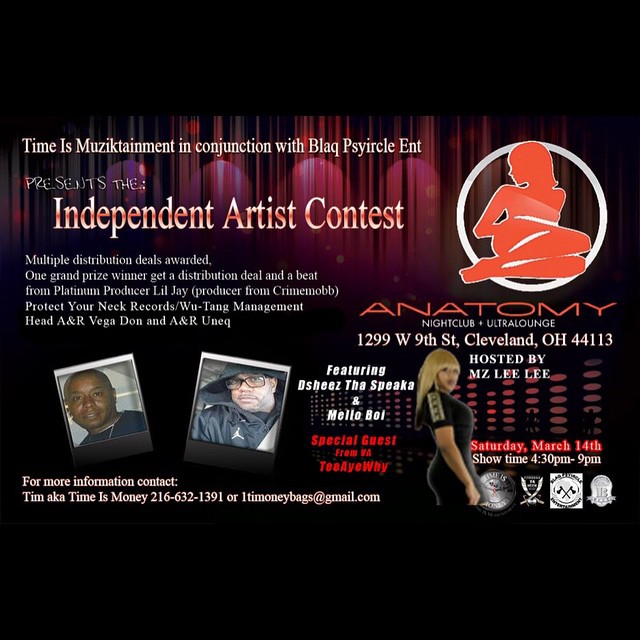The poster advertises an "Independent Artist Contest" hosted by Anatomy Nightclub & Ultra Lounge in Cleveland, Ohio, on Saturday, March 14th, from 4:30 PM to 9 PM. The event is presented by "Time is Muziktainment" in collaboration with "Blaq Psycircle Ent." The grand prize winner will receive a distribution deal and a beat from platinum producer Lil J, known for his work with Crime Mob, Protect Ya Neck Records, and Wu-Tang Management. Key figures involved in the event include head A&R Vega Don and A&R U&EQ. The poster features images of two Black men presented as Polaroid-style photographs, likely the contest participants or organizers. Additionally, there are promotional pictures of special guests D’She’s The SpeakA and Mellow Boy, and a silhouette of a provocative woman in the top right corner. Contact information, including a phone number and an email address, are provided for further inquiries. The background of the poster is adorned with red velvet curtains, enhancing its visual appeal.